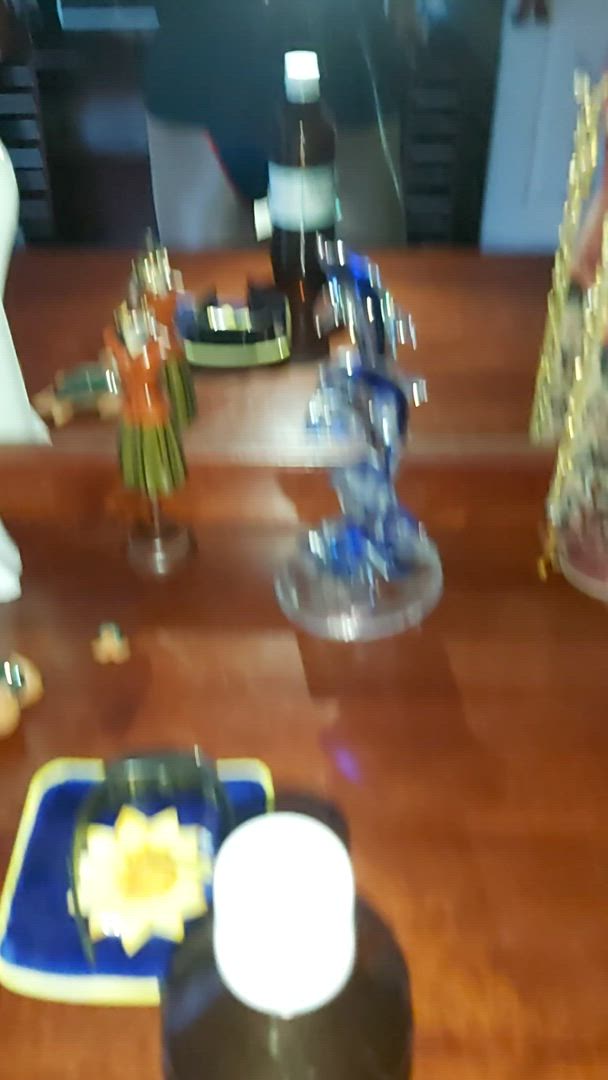The image depicts a slightly blurry but vibrant scene of a wooden table at what appears to be a casual gathering or party. Central to the composition is a striking glass bong with blue and clear elements, possibly adorned with dolphins. Scattered around the bong are various interesting items: a small cup featuring a dandelion design sits atop a coaster, giving a touch of whimsy. Nearby, there's a brown bottle with a white lid, reminiscent of those used for hydrogen peroxide, adding an intriguing, almost medicinal flair. Another brown glass bottle with a white label and cap further populates the table, suggesting beverages of some sort. To the left of the bong stands a small, captivating figurine, adding a unique decorative element to the setup. The table itself showcases a rich wood grain, grounding the eclectic assortment of items in an inviting atmosphere.